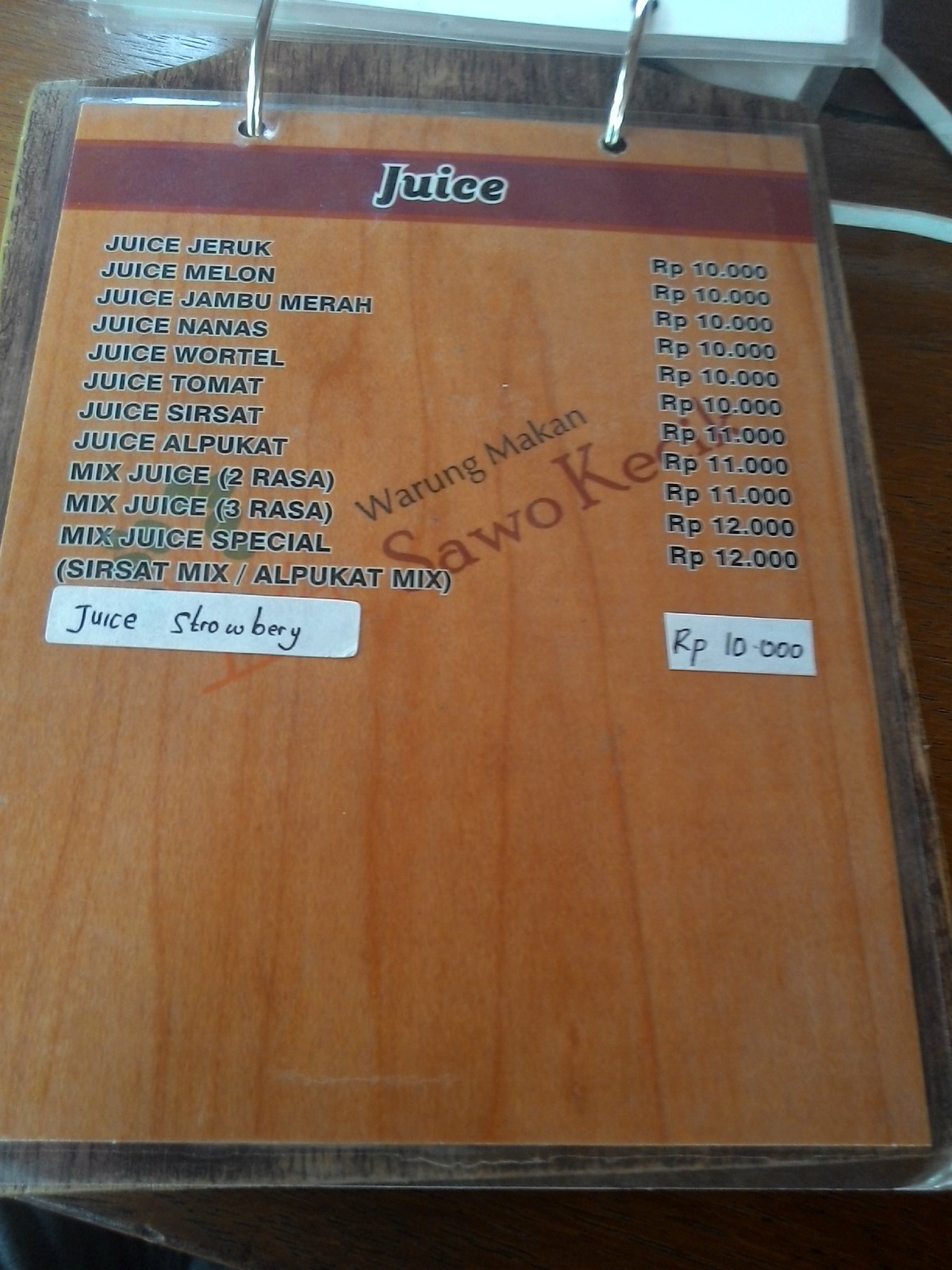This image captures a detailed juice menu, likely from an Indonesian restaurant, as indicated by the prices listed in rupiah (RP 10,000 to 12,000). The menu page is laminated and attached to a ring clipboard, suggesting it might be a take-out menu. Dominating the top is a red stripe with the word "Juice" boldly outlined in black letters. Below, there are various types of juices listed in Indonesian, including Juice Jeruk, Juice Melon, Juice Jambu Mera, Juice Non, Juice Wartel, Juice Tomat, Juice Sirsot, Juice Alpukat, Mix Juice (labeled as "2 Rasa Mix Juice" and "3 Rasa Mix Juice Special"), and a special entry, "Sirsot Mix / Alpukat Mix," written in parentheses. An additional white label, seemingly added later, lists "Juice Strawberry." The background subtly features partial words hinting at the restaurant's name, "Warung Makan Sawo," partially obscured by the prices on the menu, all printed on a faux wood texture that adds a rustic touch.